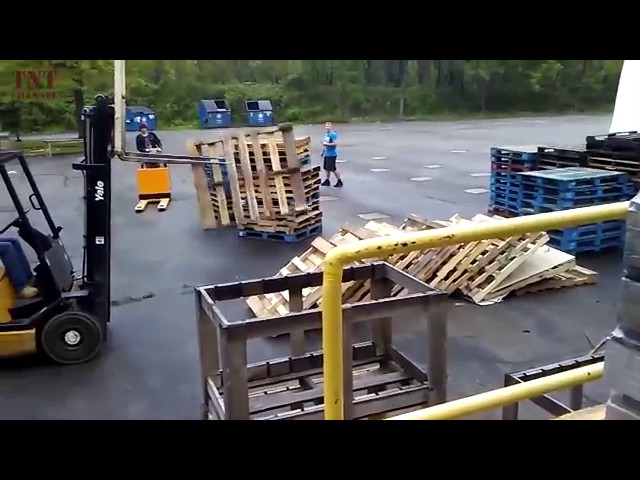The image captures a bustling construction area within a parking lot, characterized by a dark gray asphalt surface. Central to the scene are several workers engaged in moving a variety of wooden pallets using different types of pallet jacks; one is manually operated while another is motorized. Additionally, a part of a yellow-railed machine lies in the lower right corner. Dominating the left side is a striking yellow crane with a black crane area. In the mid-ground, a black brick wall supports a metal framework container. On the far right, numerous stacks of wooden baseboards and blue-colored panels are visible, some of which appear toppled over. In the distance, large blue dumpsters are positioned against a backdrop of lush green trees. Also notable is a logo in the upper left corner with the text "TNT" in maroon, accompanied by another indecipherable red word beneath it. Black rectangular bars at the top and bottom frame the image, suggesting it might be a screenshot from a video.